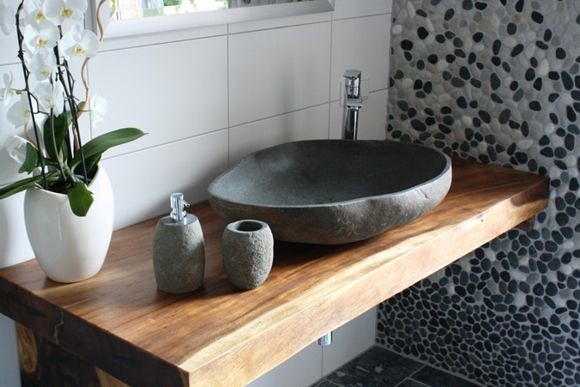The image showcases an artistic and rustic sink setup. The backdrop features large, white tiles with clear grout, providing a clean and minimalistic contrast to the elaborate sink area. Positioned above the sink is a white-framed mirror. The wall to the right is adorned with a speckled stone pattern in black, white, and gray, arranged in a loose spiral design centered around the sink. The flooring consists of black tiles, and part of the silver piping beneath the sink is visible.

The sink itself is mounted on a medium brown wooden table, likely treated to resist water damage. Atop the sink's surface sits a white vase filled with white orchids, adding a touch of elegance with their realistic or artificial appearance. Adjacent to the vase, there's a soap dispenser that resembles a gray stone, maintaining the natural aesthetic. Next to the dispenser is another gray stone-like container, presumably for holding toothbrushes.

The sink basin, raised above the wooden table, looks as though it’s carved from a large rock, adding to the natural, rustic theme. The sleek, single-handle silver faucet integrated into the spout gives the setup a trendy, modern touch. This detailed composition combines natural elements with contemporary design, creating a stylish and unique bathroom fixture.